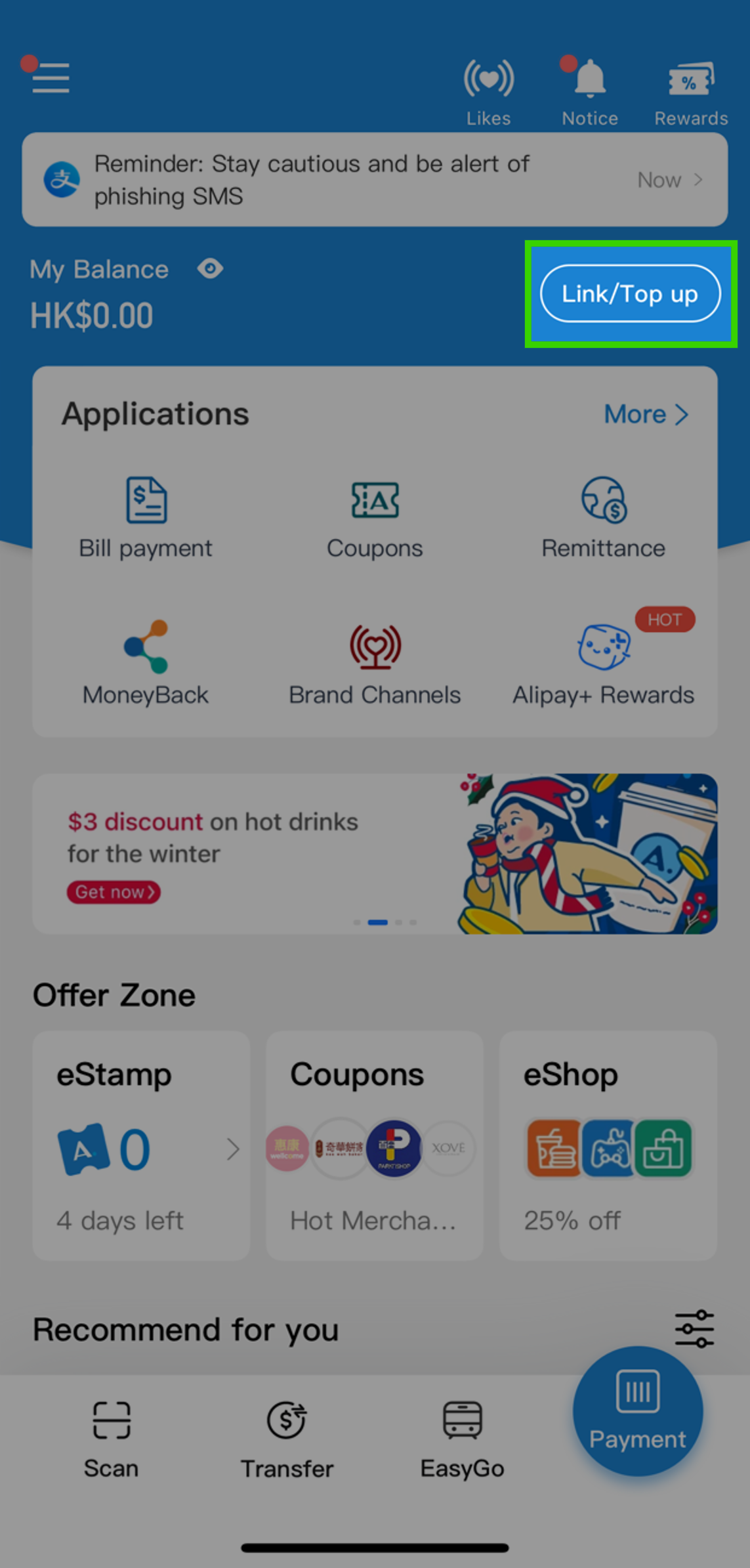Top left corner features a red dot notification with a bell icon—suggested for users who appreciate timely alerts. In this section, users can find rewards, place reminders, take cautions, and stay updated on shows.

Below that, there is a balance overview area denoted as "My Balance." Notably highlighted in this area is "HKS" with a green and blue center. This section also contains important application features including options for bill payment, coupons, remittance, and money back. 

A section labeled "Brand Channels" follows, featuring icons and options such as "Alley," "Play," and "Plus Rewards." 

Another visually engaging portion showcases cubes and a cow, with a central red oval labeled "Hot." The text within a window here reads, "$3 discount on hot drinks for the winter."

The image prominently features a woman running away with a Santa hat, carrying a warm drink with a background inclusive of a coffee cup and glittering stars. 

There is also a designated "Offer Zone" with an e-stamp, marked with the letter "A" and a notice that there are zero to four days left for certain coupons. Additional sections include an "e-Shop" with color indicators in orange, blue, and green, marked as "24 South."

Further at the bottom of the image, recommendations labeled "For You," options to scan, transfer, and easy go functionalities, and blue payment information are presented.

Overall, the image is a dynamic and busy collage of offers, alerts, and functionalities, providing an engaging and interactive user experience.